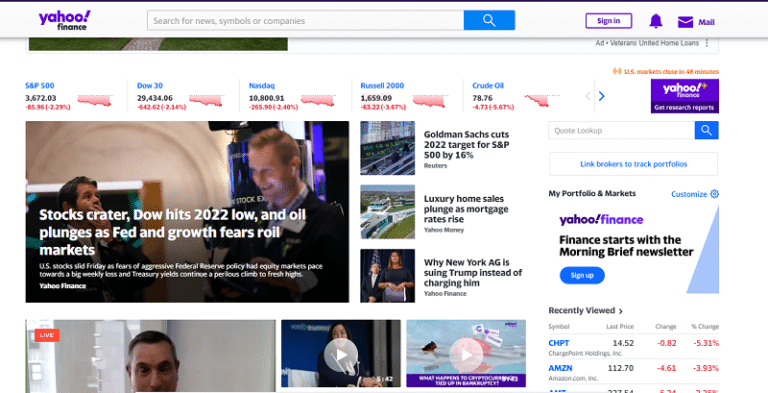This screenshot captures the upper portion of the Yahoo Finance website. In the top left corner, the iconic Yahoo logo in purple is prominently displayed, complete with its distinctive exclamation point. Directly below, "Finance" is written in a sleek black font. Adjacent to this is a long, rectangular search box featuring a blue square with a magnifying glass icon, symbolizing search functionality. To the right of the search box is a sign-in button, flanked by a small purple bell icon.

Further to the right, a purple envelope icon appears next to the word "Mail," forming part of the top navigation bar. The web page itself is populated with various colored images, mainly showcasing people. One notable image box contains a photograph of two white men. Below this, another box depicts a single man. Adjacent to that is a box displaying what looks like a video featuring a woman. Next to this video, another box contains what seems to be a cartoon image, also in video format, adding a whimsical touch to the page.

Directly beneath the Yahoo Finance logo is a horizontal bar that provides real-time stock market indices, showcasing percentages and figures for prominent markets like the S&P 500, the Dow, and the NASDAQ. This comprehensive top section effectively blends multimedia elements with financial information, offering a rich user experience.